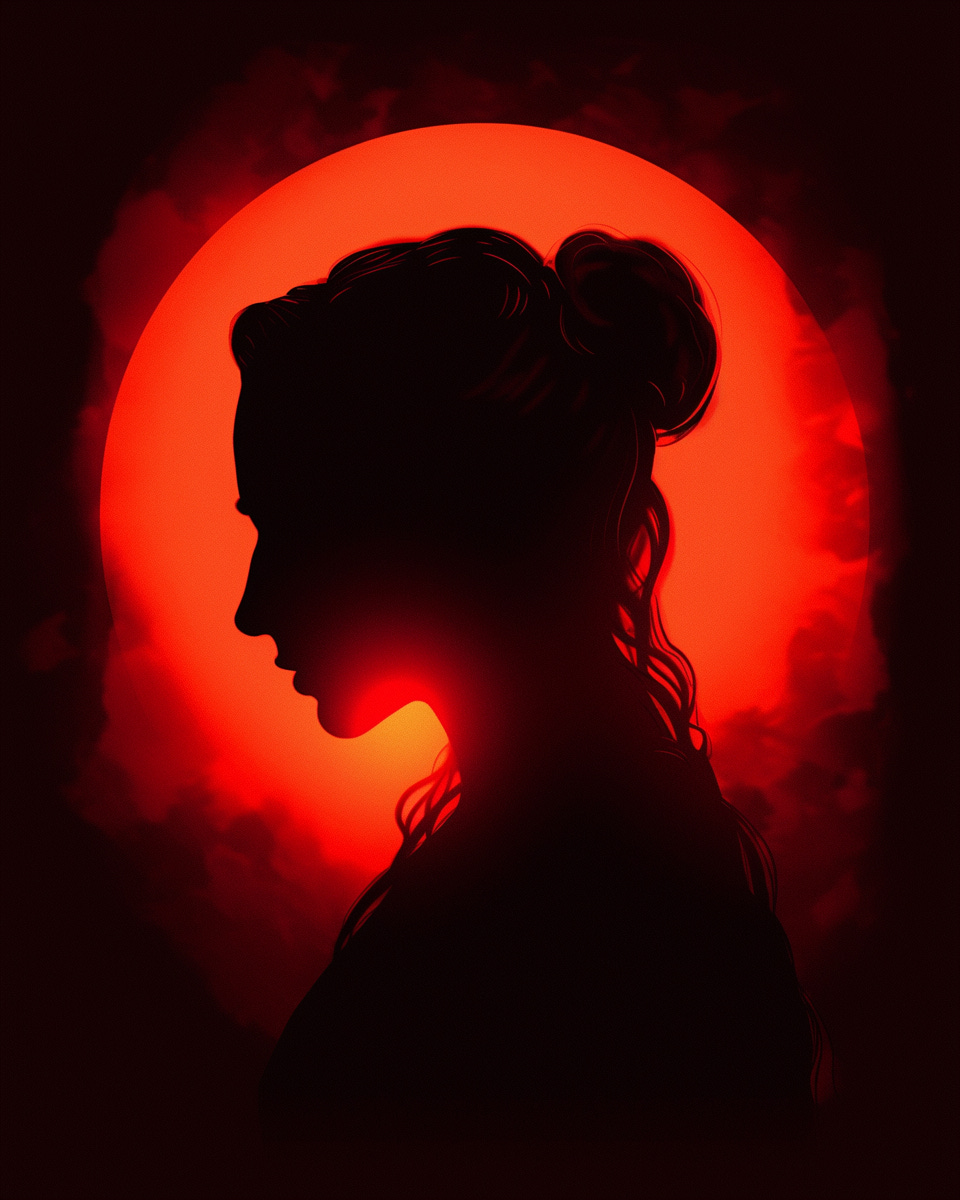The image portrays the side profile silhouette of a woman, created either through AI generation or as a painting. The woman has long, curly hair, primarily tied up in a bun, with some strands draping down the right side of her neck and back. She appears to be gazing thoughtfully or concerned towards the lower left corner of the image. Prominent features such as her sharp jawline, defined chin, and somewhat larger nose and lips are clearly outlined. The background features a large red-orange circle, resembling the moon or sun, with surrounding splotches mimicking clouds, steam, or smoke. The silhouetted figure and background contrast starkly, with the glowing circle casting a yellowish to reddish light beneath her chin and against her neck.